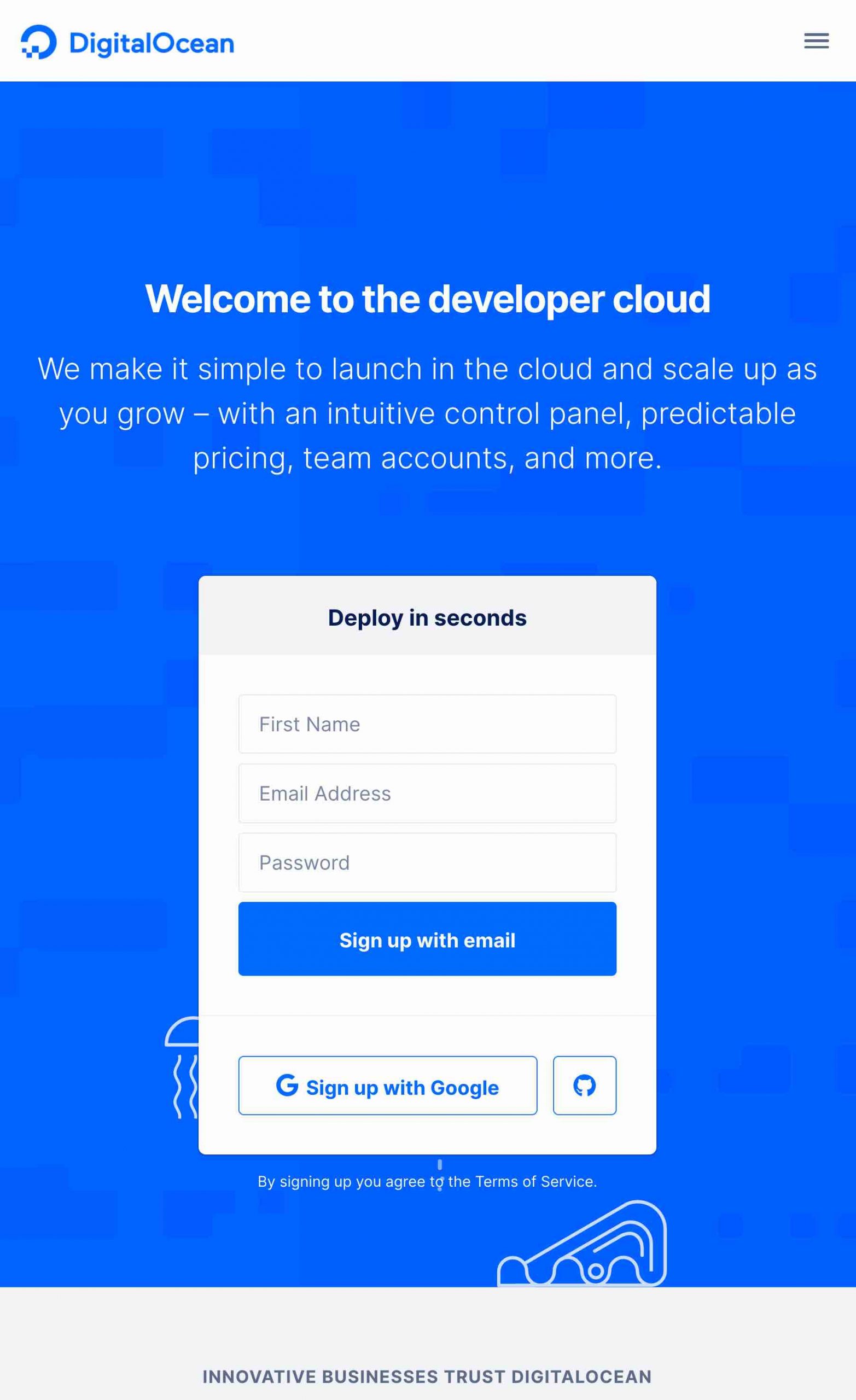This image showcases a screenshot of the DigitalOcean app interface. At the top left corner, the app name "DigitalOcean" is displayed in blue, accompanied by a pixelated, blue 'O' symbol. The top right corner features a gray tab button. Below this, there is a prominent blue box with blocky ink blue and sky blue patterns. Inside the blue box, white text welcomes users with the message: "Welcome to the Developer Cloud. We make it simple to launch in the cloud and scale up as you grow with an intuitive control panel, predictable pricing, team accounts, and more."

Further down, a white section is dedicated to new user registration. This section includes fields for "First Name," "Email Address," and "Password" followed by a blue "Sign Up with Email" button. Additional options include a button to sign up with Google and another adjacent button. Below these, the image reminds users that by signing up, they agree to the terms of service. Lastly, a note at the bottom reassures users with "Innovative businesses trust DigitalOcean."